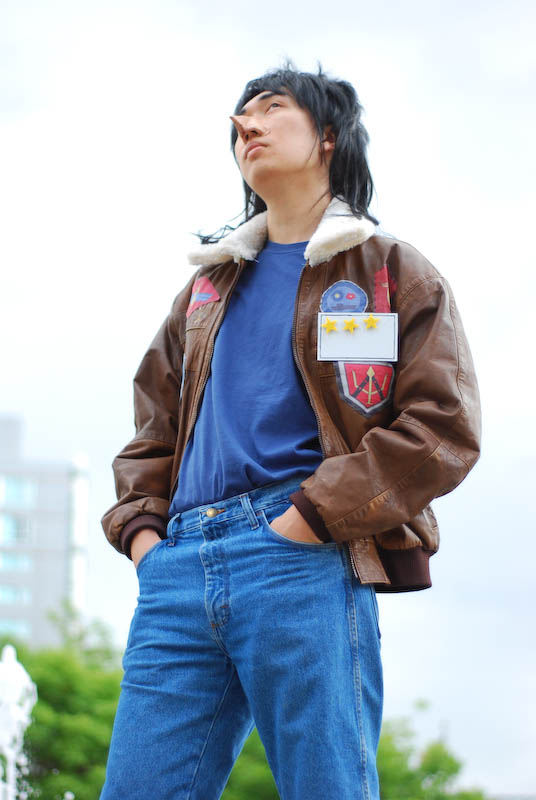The image depicts a young Asian man standing outdoors in a city-like environment. The photographer's perspective is from below, capturing the man from about thigh level to the top of his shaggy, long, dark hair that has an unkempt appearance. He is dressed in blue jeans and a navy blue t-shirt, paired with an unzipped brown bomber jacket adorned with numerous patches. His hands are casually in his pockets, and he stands with a demeanor that suggests disinterest or boredom, as he gazes slightly upward into the blue sky, dotted with clouds. His nose is noticeably altered, extended by a prosthetic that makes it look unusually pointy, akin to an elf's nose. A distinct feature of his outfit is a white tag with three yellow stars attached to the left breast of his jacket, resembling a name tag but devoid of any name. Behind him, the background shows green trees and a large multi-story building with numerous windows, contributing to the urban atmosphere.